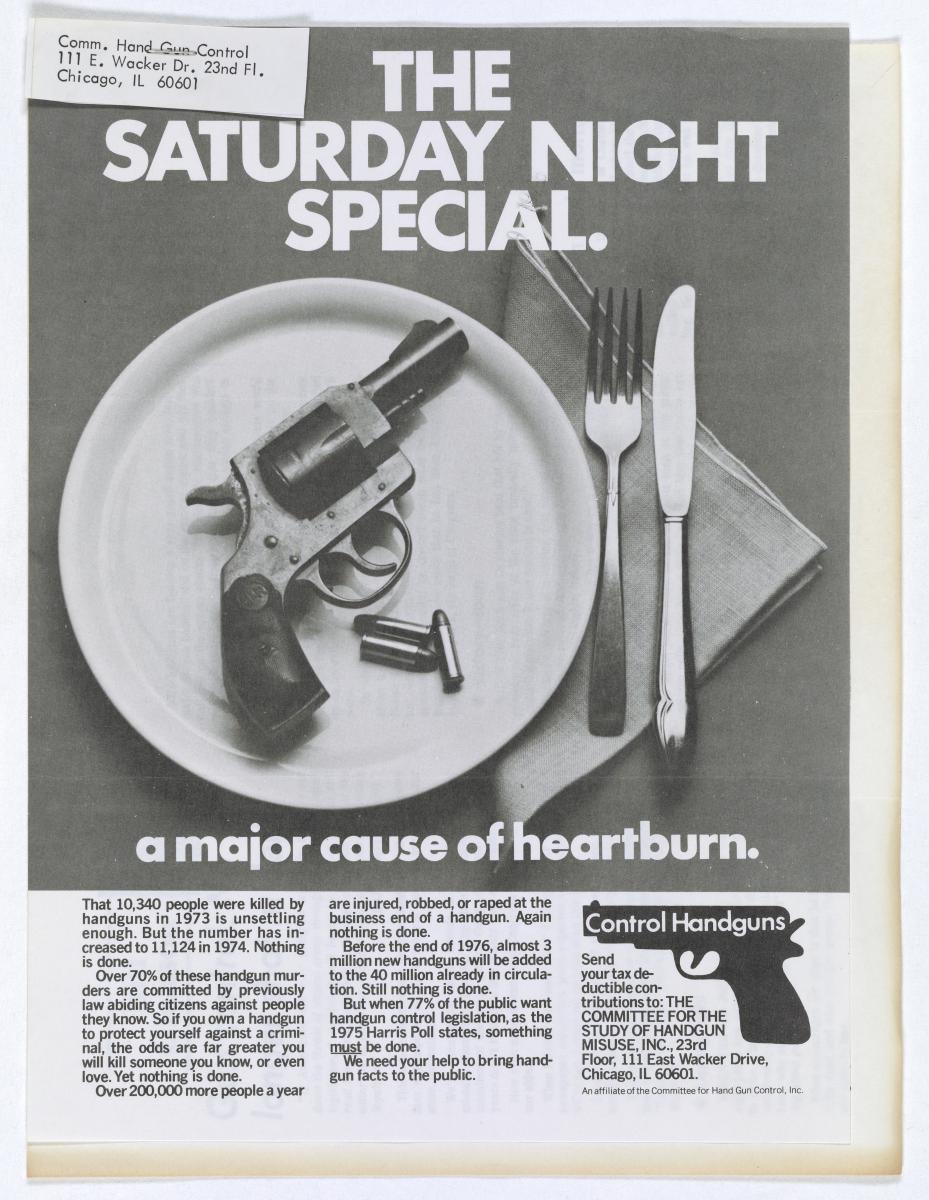The image is a detailed magazine page or flyer featuring a provocative layout to highlight handgun violence. At the top of the page, in stark white letters, it reads "The Saturday Night Special." Central to the image is a white circular plate with a short-barrel handgun and three bullets placed on it. To the right of the plate, a neatly folded napkin lies beneath a fork and knife, enhancing the table setting visual. Beneath this striking visual, the text in white letters states, "A major cause of heartburn." Further down, the article reveals unsettling statistics: 10,340 people were killed by handguns in 1973, a number that increased to 11,124 in 1974, with the grim note that nothing has been done to address it.